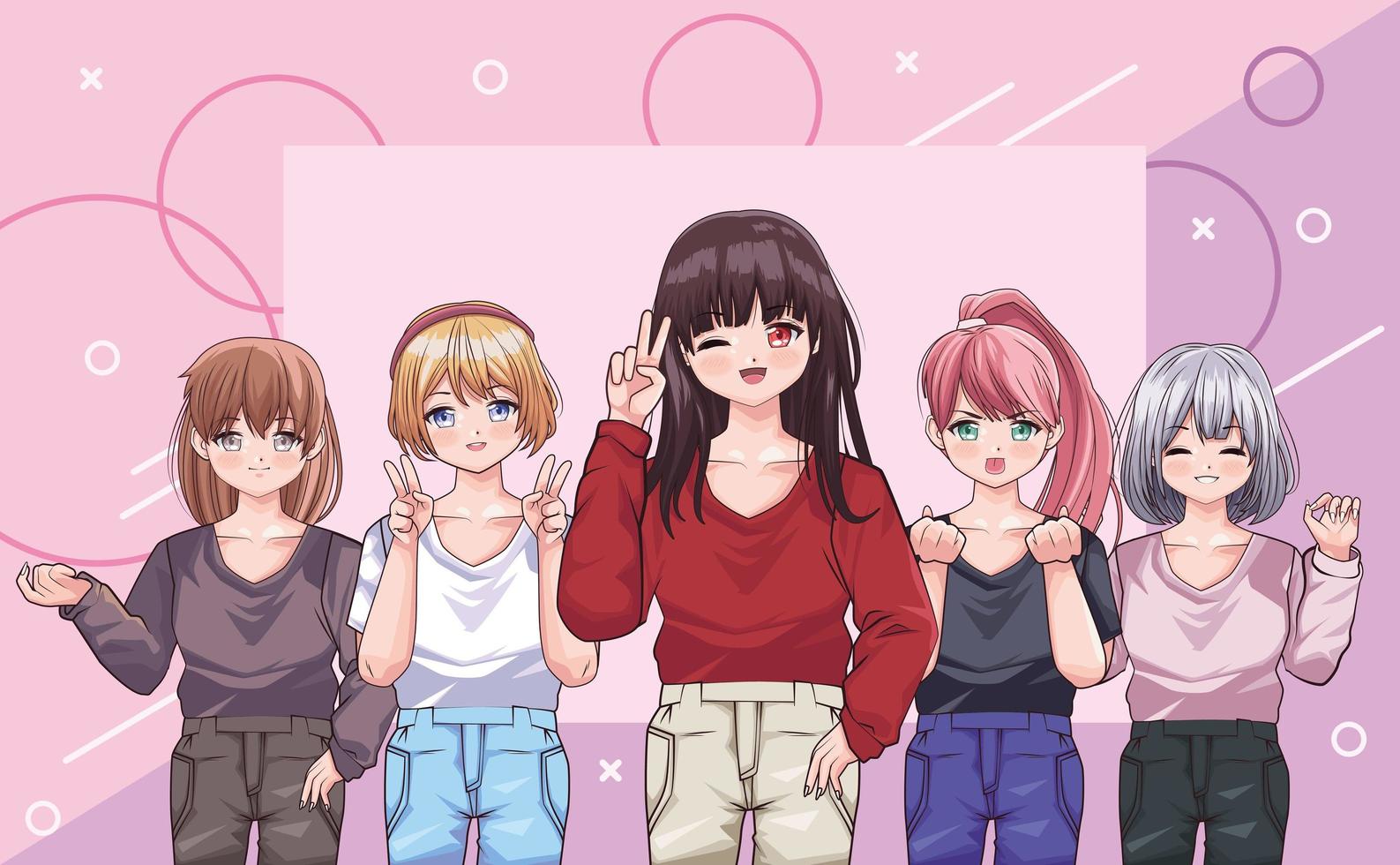In this detailed anime-style graphic, five young girls stand against a vibrant pink backdrop that varies in tone from lighter purple hues to brighter pink shades, framing the characters prominently. The image is notably wider than it is tall, making it ideal for a feature on a website or news article. The girls, each sporting big eyes and distinct hairstyles, exude a cutesy charm reminiscent of manga or anime art. Despite having similar builds, their hair colors are diverse: light brown, blonde, dark brown, salmon pink, and silvery gray.

From left to right, the first girl has light brown hair and wears a deep purple top paired with green trousers. Her pose is confident, with her right arm raised at the elbow and her left hand resting on her hip. Next to her, the blonde girl has a short haircut adorned with a dark ribbon. She dons a white loose-fitting top and light blue trousers. The central figure, the tallest among them, has dark almost-black hair with bangs and is winking playfully. She strikes a peace sign with her right hand and rests her left hand on her hip, wearing khaki-colored jeans.

Moving further right, the fourth girl sports salmon-colored hair tied in a ponytail that cascades over her left shoulder. She wears a dark top, possibly black or dark gray, with purple pants, and her hands are raised in fists near her shoulders. The final girl has silvery gray hair and closes her eyes with a gentle smile. Her left arm is raised in a slight wave, while her right arm is obscured behind the penultimate girl. She is dressed in a light mauve-colored top and green trousers.

Their cohesive yet individualistic clothing style suggests they might be a young pop group, each member dressed in a similarly designed outfit but in different colors. The harmonized yet varied attire and hairstyles enhance their collective yet distinct personas, set against the eye-catching pink and purple circular backdrop that adds depth and focus to the ensemble.